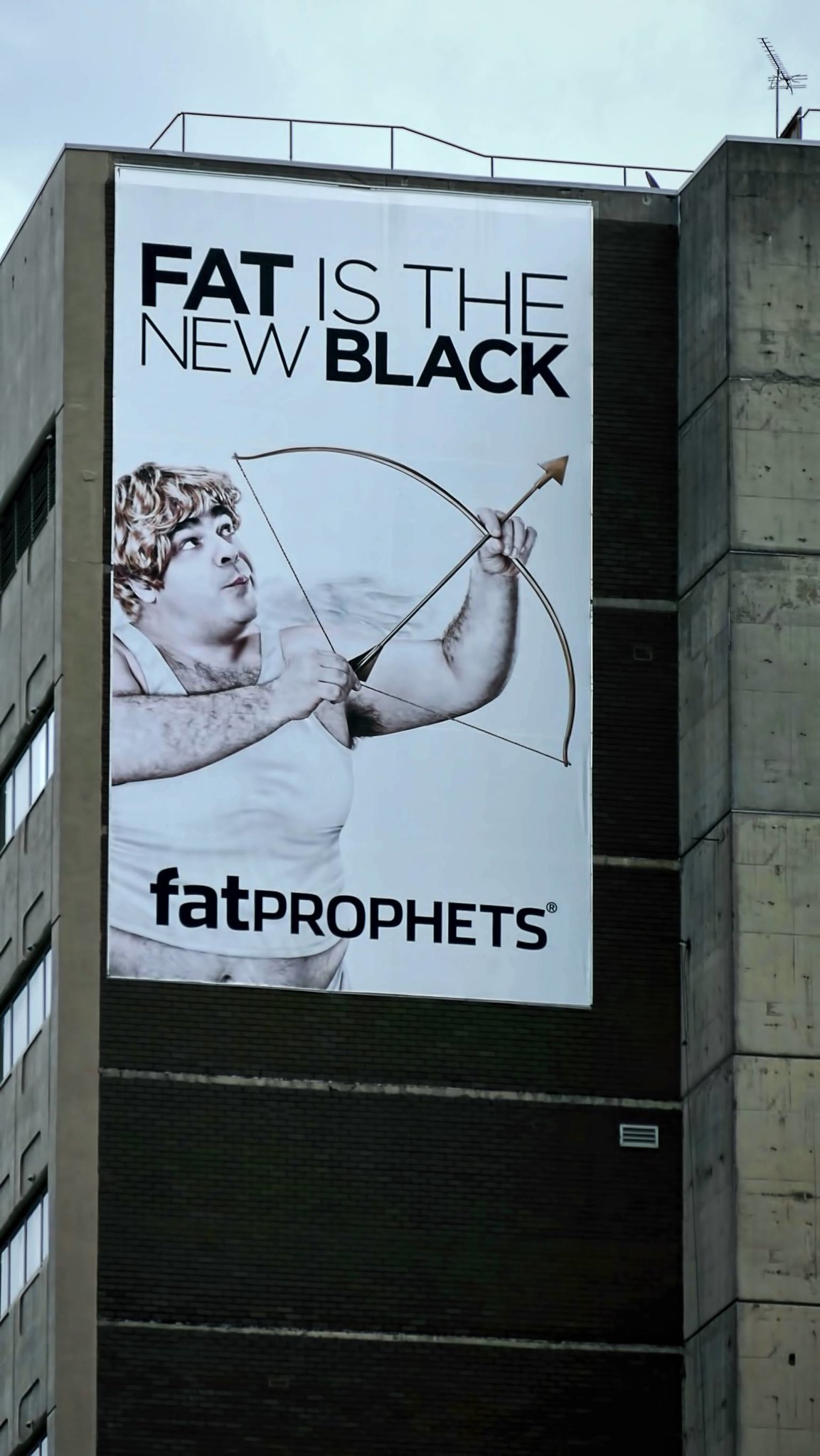In this photograph, a towering stone building captured from below dominates the frame. The rooftop is bordered by a metal railing encircling its perimeter. A large white banner, spanning three floors in height, is prominently displayed on the building's facade. The banner bears the slogan "FAD is the new black," and features an image of a hefty man dressed as Cupid. This comedic Cupid is wearing a white tank top, commonly known as a 'wife beater,' which exposes his protruding belly. In his hands, he brandishes a bow and arrow. Below the image, the text reads "Fat Prophets." On the left side of the building, rows of windows are visible on each floor, segmented by large black stripes running horizontally across the structure at each level. Just beneath the poster, a white metal vent is apparent, integrated into the building’s exterior.